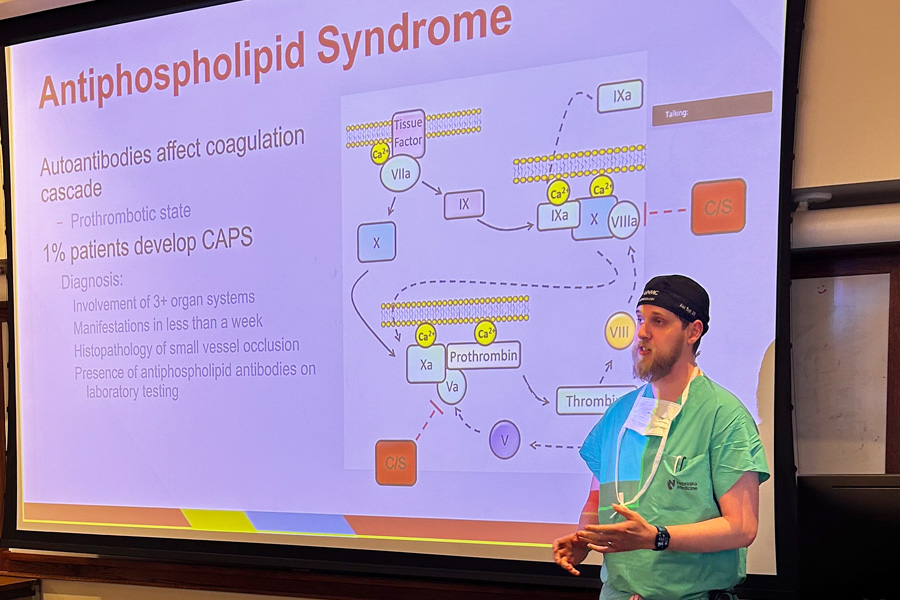The photograph features a man likely in his 30s, dressed in light blue scrubs with a white medical mask hanging around his neck and a black hat containing his hair. He has a beard and a black watch on his right wrist. The man appears to be a medical professional, potentially a doctor, as he is giving a presentation. He stands in front of a large screen that prominently displays information about Antiphospholipid Syndrome. The screen includes detailed text such as "Auto-antibodies affect coagulation cascade – prothrombotic state," "1% patients develop CAPS (Catastrophic Antiphospholipid Syndrome)," "Diagnosis: involvement of three or more organ systems," "Manifestations in less than a week," "Histopathology: small vessel occlusion," and "Presence of antiphospholipid antibodies on laboratory testing." Additionally, there is a complex medical diagram with various labels like "tissue factor" and "VLA-X, IX, IXA-X," as well as numerous arrows illustrating the pathway of the syndrome. The man is captured mid-sentence, emphasizing his active engagement in explaining the medical content.